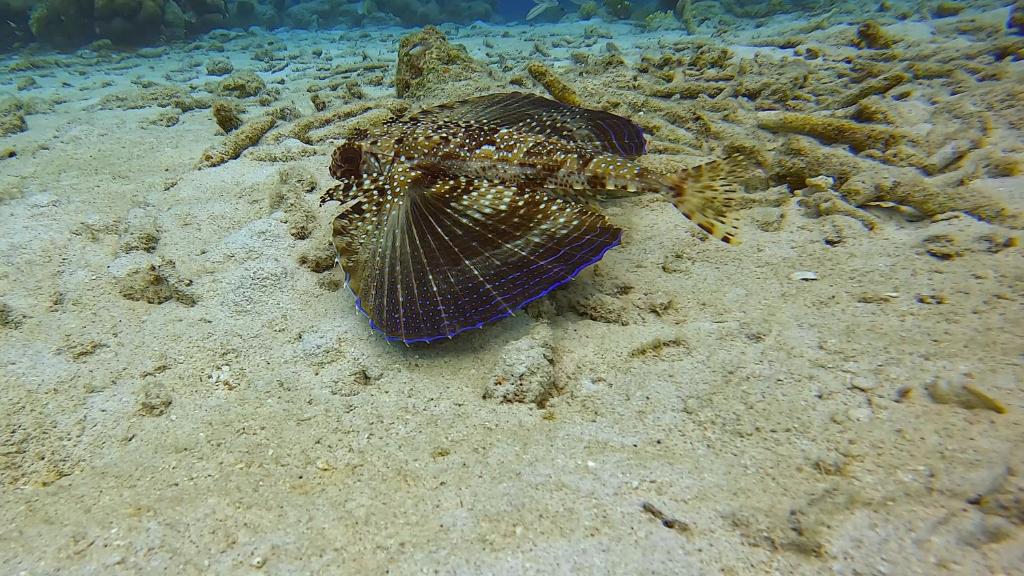An intricate and vividly detailed underwater scene showcases a unique marine creature resembling a butterfly or angel fish, set against a light brown, sandy ocean floor scattered with barnacle-like formations that resemble corn cobs. The creature dominates the center of the image, its delicate, wing-like fins spread wide with striking electric blue edges that transition into a dark blue trim. Closer to the body, white dots speckle the predominantly brown fins, blending seamlessly with the light brown seafloor below. Its head appears as a dark, almost black ball on the left, subtly camouflaging amidst the environment. The background features hues of dark and light blue, accentuating the vibrant colors and intricate patterns of the fish, which include lines and spots adding to its camouflage effect. The overall setting is a serene underwater landscape that hints at both the beauty and subtle complexity of marine life.